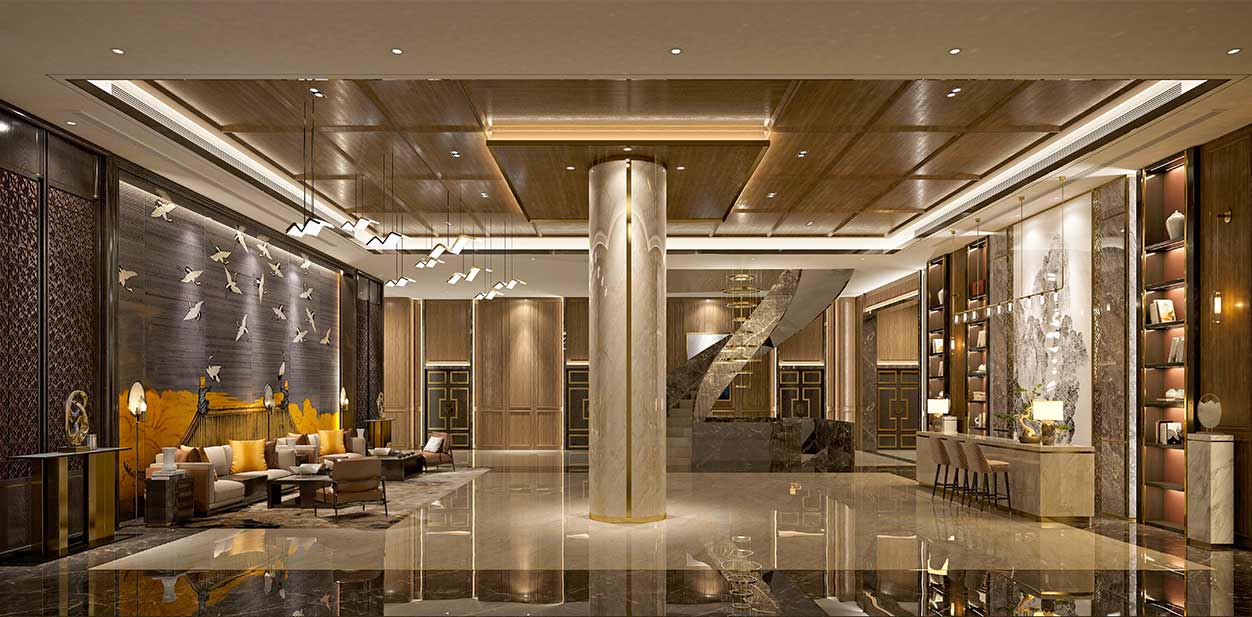The photograph depicts a luxurious lobby, likely in a high-end hotel, characterized by its cavernous and expansive design. Dominating the ceiling is an exquisite art installation resembling birds in flight. This installation is complemented by a large, visually striking painting on the wall, which also features birds soaring in various directions against a backdrop with yellow hues at the bottom. In front of this painting, there is a well-appointed seating area that includes a sofa, a coffee table, and several chairs with many pillows, offering a cozy yet elegant spot for relaxation.

The floor, made of highly polished marble, reflects the room's ample lighting and contributes to the overall sense of opulence. A prominent, round column, ascending from floor to ceiling, adds architectural interest; it is adorned with square lights at the top, enhancing the room's modern aesthetic. The lobby also features tall, slender lamps and additional pieces of abstract art displayed on side tables.

On the right side of the image, there is a sophisticated bar-like area with a wooden countertop and several light-colored chairs. This section is well-lit, with shelves showcasing vases, pottery, and books, furthering the ambiance of refinement. Decorative track lighting and gold accents contribute to the room’s warm and earthy color palette. In the background, a spiraling staircase adds a dynamic element to the space, indicative of the meticulous attention to design and detail that pervades this luxurious environment.